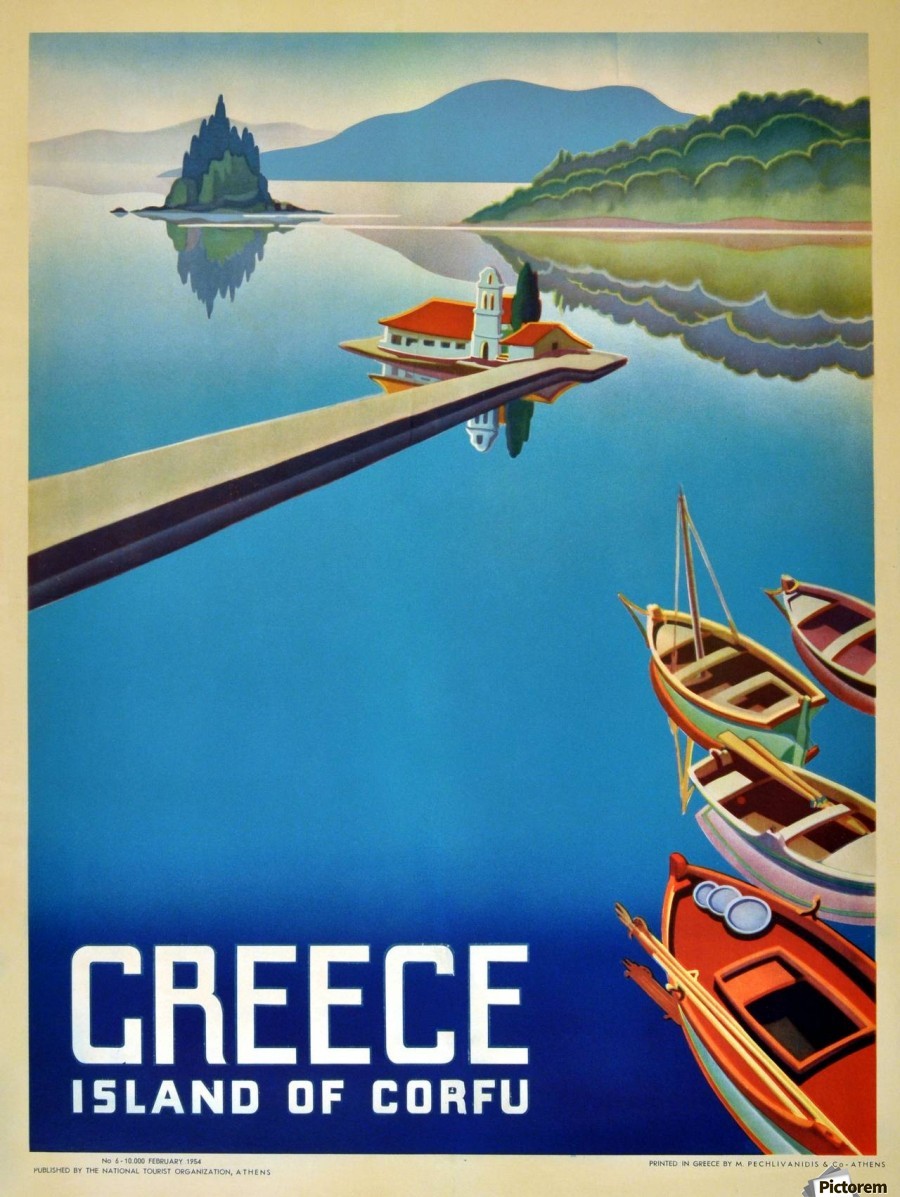This promotional poster for the Greek island of Corfu depicts a serene scene centered around a large, strikingly blue lake. Dominating the lake is a small floating home with a red-orange roof. The home features a prominent three-story, round structure and a smaller adjoining structure, surrounded by a green tree. Leading from the shore to this floating home is a long boardwalk that appears to be wooden.

In the foreground, four vividly colored sailboats—orange, white, green, and pink—are seen, each with benches and paddles, and their sails down, highlighting their rowboat style. These boats are sailing towards the boardwalk, suggesting an invitation to explore the tableau. 

The background is adorned with lush green islands and towering silhouettes of blue mountains, echoing the deep blue of the water. The scene is framed by text on the lower left corner of the poster which reads, "Greece, Island of Corfu," reinforcing the image as a travel advertisement. This detailed and vibrant portrayal invites viewers to imagine themselves visiting the scenic island, partaking in leisurely boating activities while soaking in the picturesque landscape.